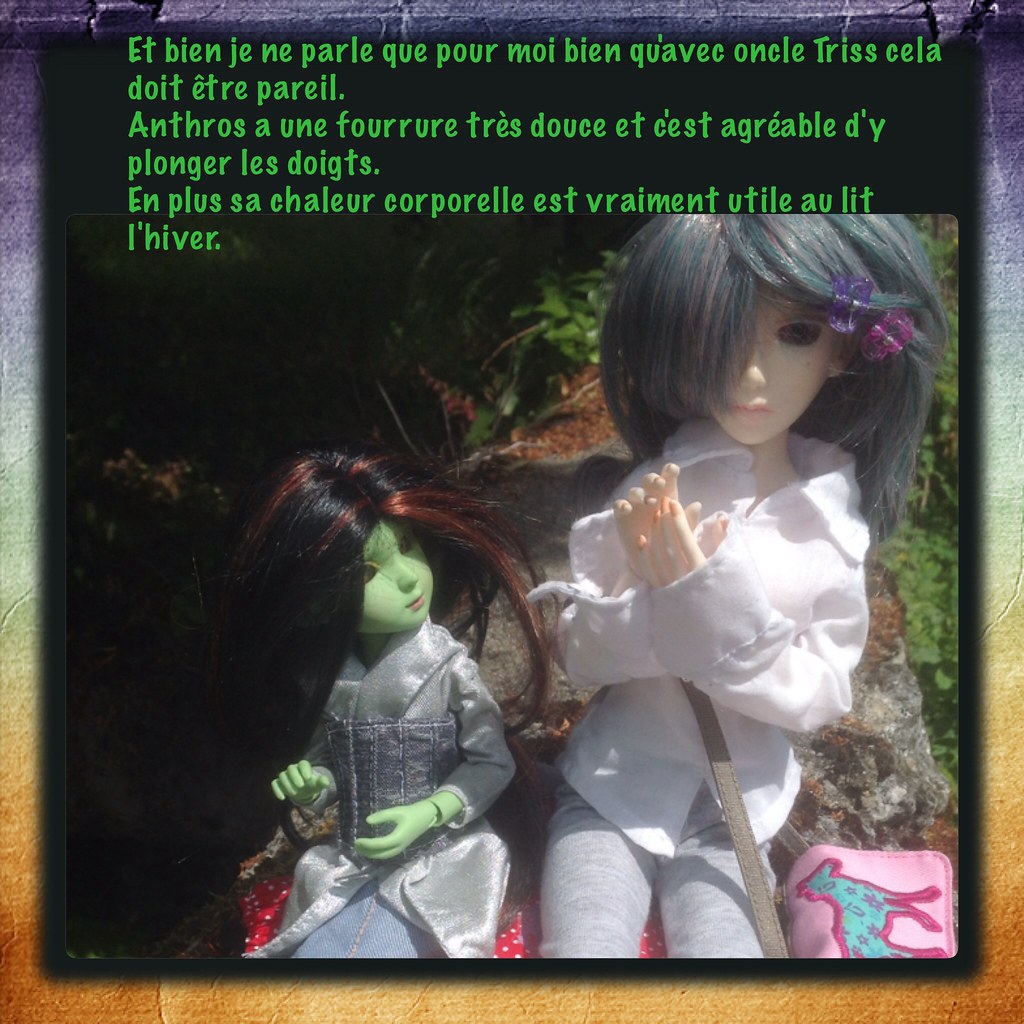The image depicts two plastic dolls sitting on a red blanket with white polka dots, set outside among some fake plants. The smaller doll on the left has green skin and black hair with reddish-brown streaks, which is styled to the left. She is dressed in a silver long coat. The larger doll on the right, wearing a light-colored top and gray leggings, sits with her hands clasped in front of her. She has greenish-purplish hair pinned with purple and pink hair clips, which partly covers her face. She also sports a pink cross-body bag with a blue horse design. Above the dolls, there is text in green font on a black background which appears to be in French.